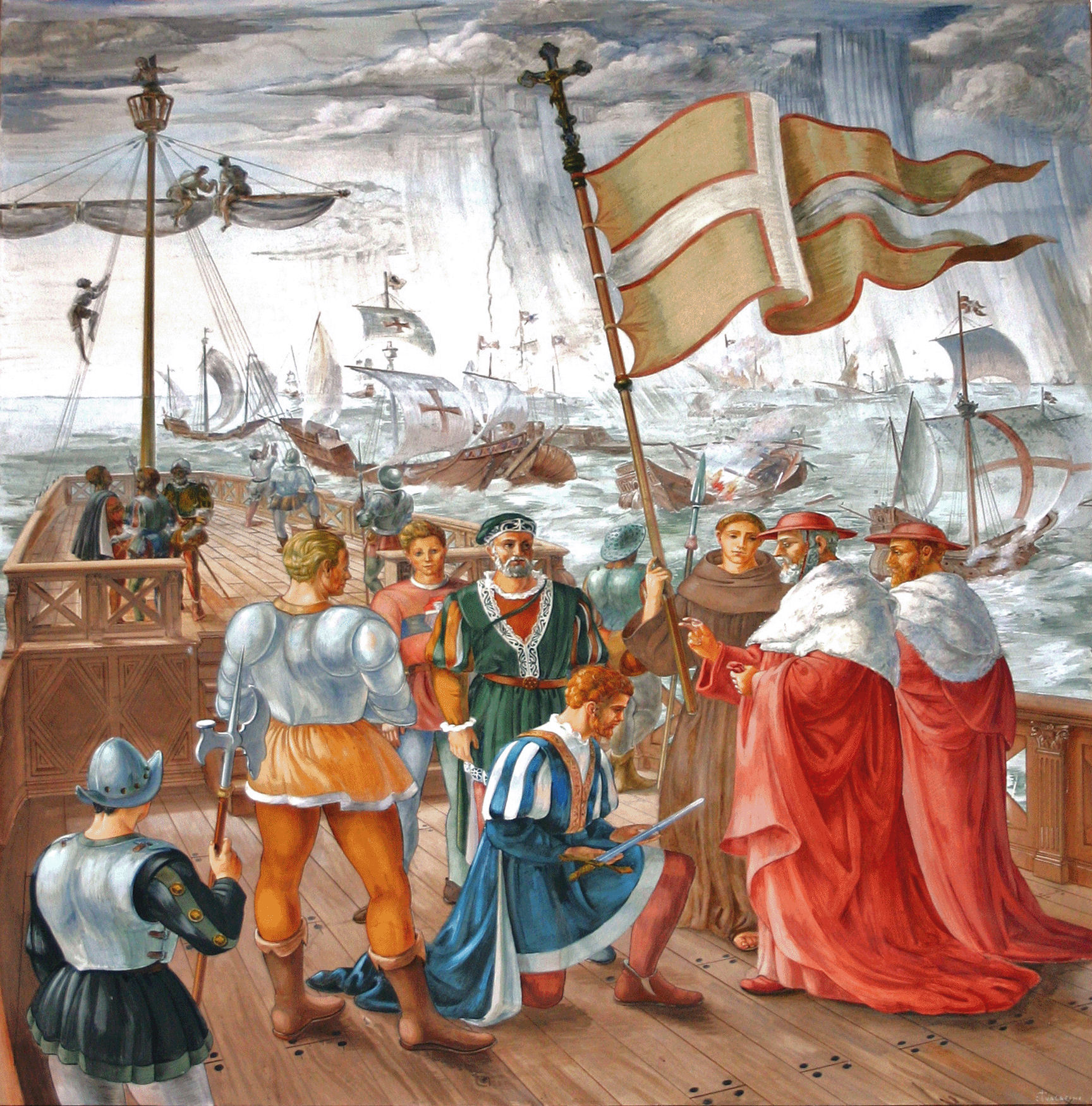This painting depicts a medieval scene on a large, brown wooden ship amidst a tumultuous sea under a gray, stormy sky. Central to the composition are several figures on the ship's deck. A cleric or priest dressed in a brown robe prominently holds a large flag adorned with a white cross. Flanking him on the right are two men in striking red robes and matching hats, each with white shawls draped over their shoulders. Kneeling before them is a man clad in a blue and white tunic with gold trim, holding a long sword, possibly in the act of being knighted. To the left, two figures in armor stand, one carrying a spear, while another man behind them grips a large axe. In the background, additional ships, some appearing distressed, float in the rough sea, with sailors climbing up the rigging and masts. Cross-bearing sails are visible amid the waves, conveying a sense of urgency and peril.